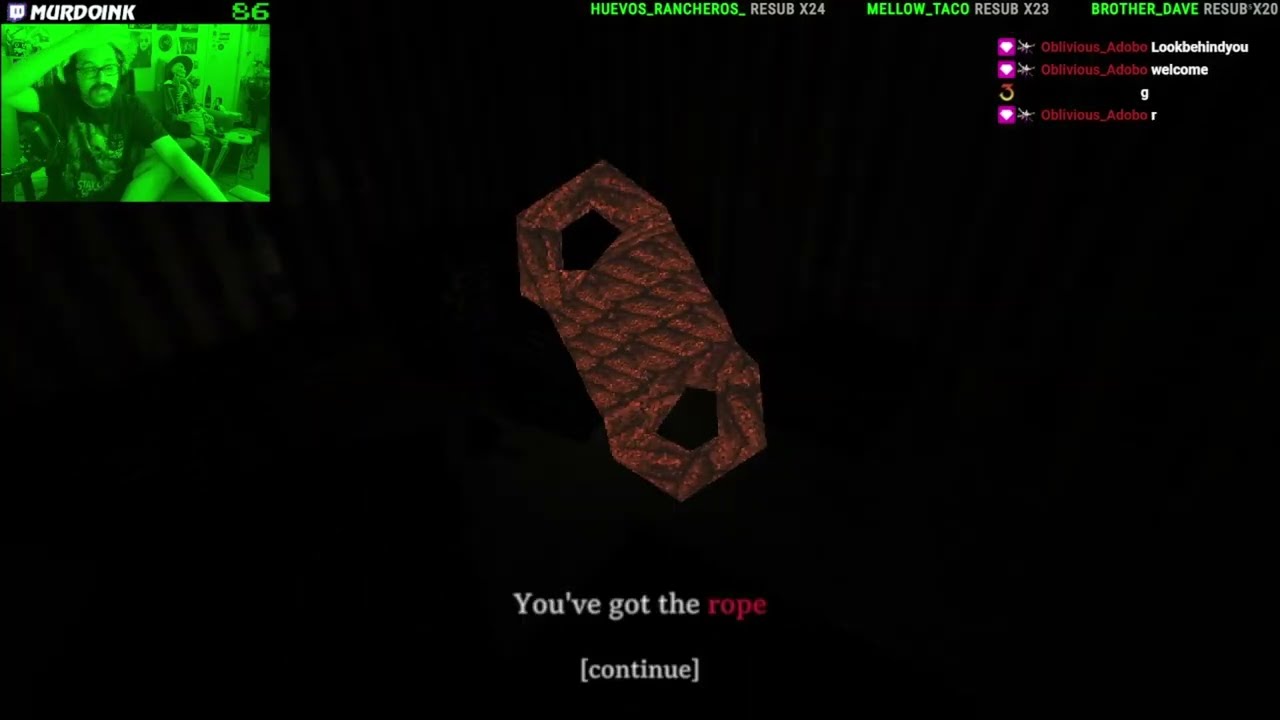In this detailed screenshot from an online video game, the main game screen occupies the center, displaying a polygonal brown rope with two loops on the top and bottom and a coiled middle, characterized by its hard edges rather than smooth curves. Overlain text beneath the image of the rope reads "you've got the rope" with the word "rope" highlighted in red, followed by a prompt to "continue" in white font.

In the upper left-hand corner, there is a webcam feed of a streamer, who appears to be a white male with a large black mustache and balding head, wearing a black t-shirt. The webcam feed has a green filter, reminiscent of night vision goggles, showing the streamer with his left arm extended in front of him and his right hand resting on his head. Above the webcam feed, the streamer's gamertag "Murdoink" is displayed, along with the number 86 indicating the viewer count.

Additionally, the screen hosts a top bar listing the usernames "Huevos Rancheros," "Mellow Taco," and "Brother Dave" in green, which are possibly the names and scores of other players. There is also game chat in the upper right corner, featuring usernames in red with corresponding text in white.